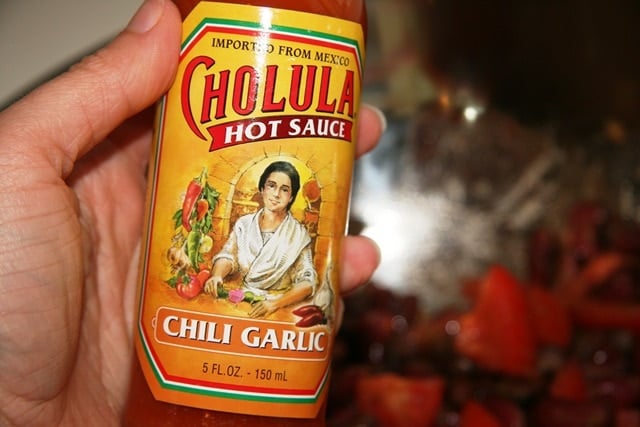This detailed landscape-format photograph features a hand emerging from the lower left side, extending towards the left center. The hand, with its palm facing forward, grips a glass bottle of hot sauce. The thumb is positioned at the edge of the bottle, while two fingers wrap securely around its back.

The bottle of hot sauce is cylindrical, adorned with a yellow label. The label design includes vibrant red, white, and green stripes along its border. Central to the label are the words, "Imported from Mexico, Cholula Hot Sauce, Chili Garlic, 5 ounces, 150 ml." Additionally, a meticulous illustration depicts a woman in a white shawl standing before an arched doorway, with a strand of chilies hanging on the wall beside her.

To the right side of the image lies an out-of-focus round object, decorated with bright red elements around its perimeter and featuring a light area in its center. This blurred element adds depth and contrast to the sharp focus of the hot sauce bottle and the gripping hand, making the bottle the undoubted focal point of the photo.